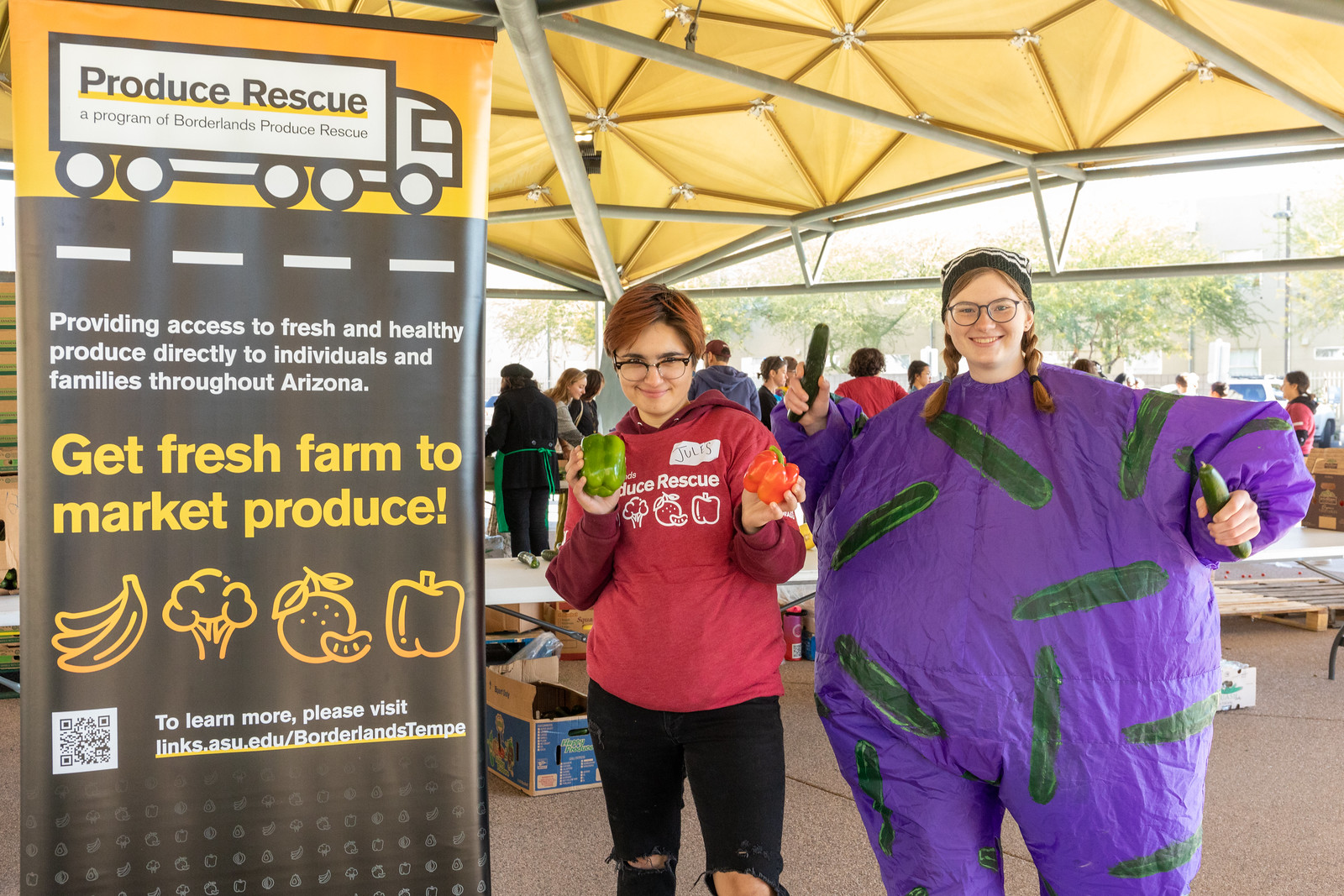The image captures a lively event scene under a tented structure with metal poles, bustling with people and tables in the background. Foregrounded are two women posing for the camera. The woman on the left sports a large, violet, puffy costume adorned with green cucumber prints and is holding either cucumbers or zucchinis. She wears glasses. Next to her, the other woman, also wearing glasses, is dressed in a red hoodie with a matching t-shirt and black pants, holding a green bell pepper in one hand and a red pepper in the other. Both women have red hair. To their left, there's a vertical banner with an orange header featuring a semi-truck and the text "Produce Rescue, a program of Borderlands Produce Rescue." Below that, on a black background, more text reads "Providing access to fresh and healthy produce directly to individuals and families through Arizona" and promotes their website and a QR code. The banner also displays images of various fruits and vegetables, including bananas, broccoli, apples, and peppers. The scene is set under a roofed construction with some trees visible in the background.